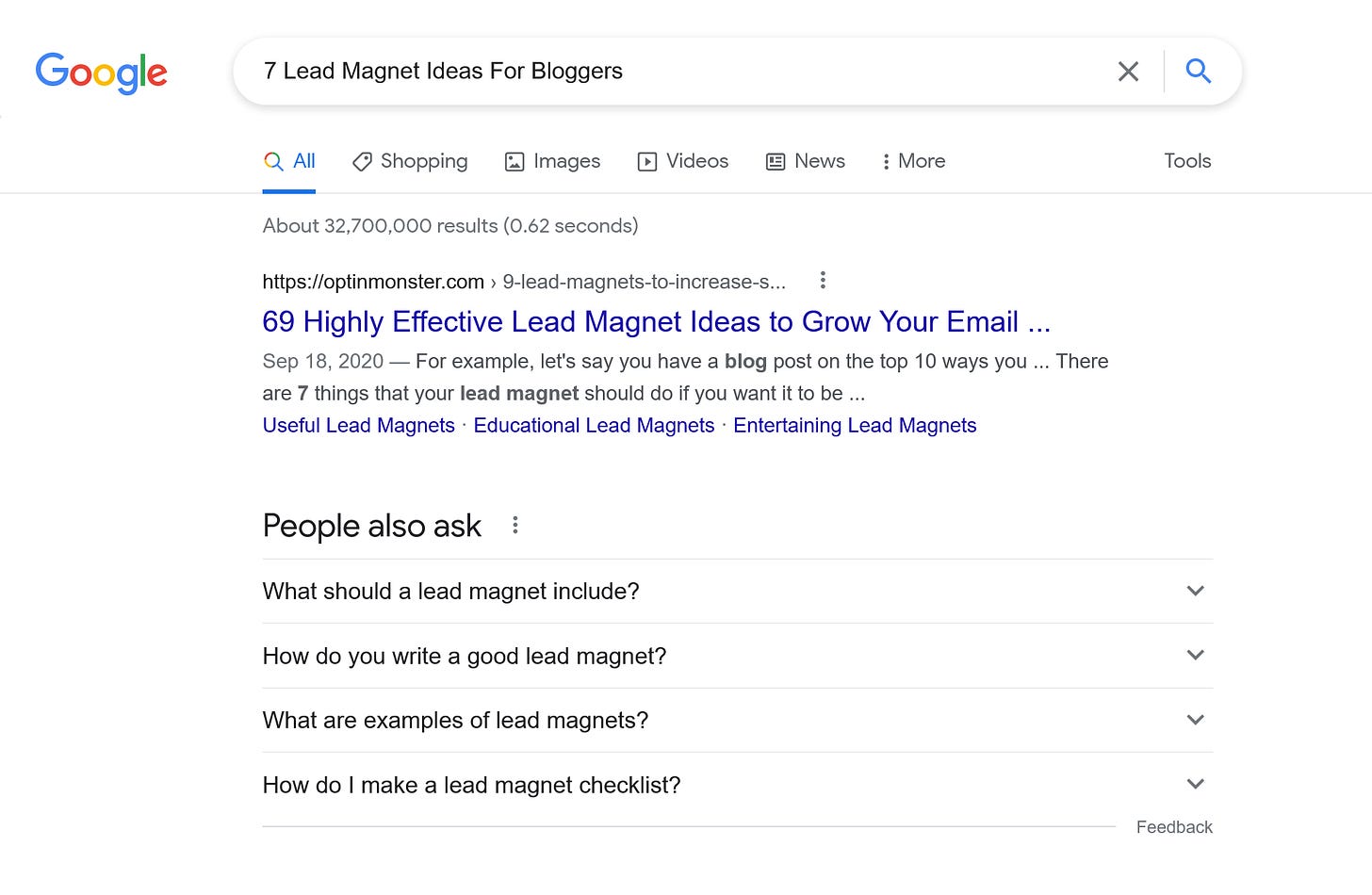The image captures a horizontally rectangular screenshot of a Google search results page. In the upper left corner, the recognizable Google logo is prominently displayed, followed to the right by an active search bar containing the query "seven lead magnet ideas for bloggers." Below the search bar, a horizontal menu offers various selection options: All, Shopping, Images, Videos, News, and More.

Directly underneath this menu, a result count states "About 32,700,000 results." The top search result is titled "69 Highly Effective Lead Magnet Ideas to Grow Your Email List," dated September 18, 2020. The snippet from this top result begins with the sentence: "For example, let's say you have a blog post on the top 10 ways you there are seven things that your lead magnet should do if you want it to be."

Further down, the "People also ask" section presents related questions such as: 
1. "What should a lead magnet include?"
2. "How do you write a good lead magnet?"
3. "What are examples of lead magnets?"
4. "How do I make a lead magnet checklist?"

In the bottom right corner of the screenshot, a "Feedback" option is visible, inviting users to provide input on the search experience.